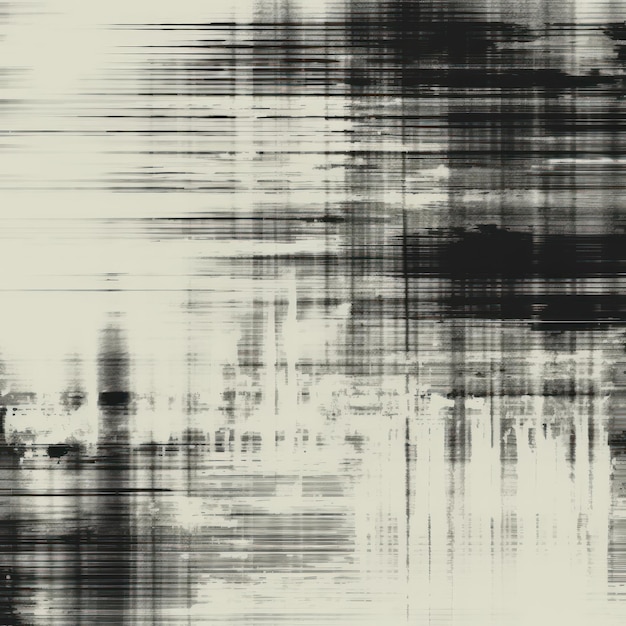This image showcases an abstract artwork in black and white, characterized by a monochrome, striped effect that resembles scratches. The horizontal black lines are dominant and dark, creating a high-contrast pattern across the image. Vertical lines are present but faded, giving a layered, textured appearance. The top section of the image features a band of thicker, dark black lines, which gradually becomes thinner and lighter towards the left side before thickening again. The bottom section has prominent white lines cutting into the black, adding complexity to the composition. The overall effect appears to be heavily manipulated, as if a photograph has been transformed into an abstract artwork or lithograph. The image evokes a sense of an outdoor scene, hinted at by a faint vertical structure in the background. The color palette includes shades of black, gray, and a desaturated yellow, enhancing the abstract, album-cover-like aesthetic.